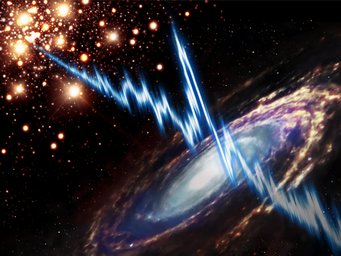The image showcases a vivid depiction of outer space with a dark, black background. Dominating the scene is a large spiral galaxy positioned slightly off-center towards the bottom right, featuring a radiant white core that transitions into hues of blue, yellow, and reddish-orange as its cloudy arms stretch out. Above the galaxy, a striking blue thunderbolt with a white center zigzags across the image from the top left to the bottom right. In the top left corner, a cluster of bright orange-yellow lights of varying sizes glows intensely at the center, becoming sparser towards the edges. The scene, likely digitally created or edited, captures a breathtaking and surreal cosmic tableau.